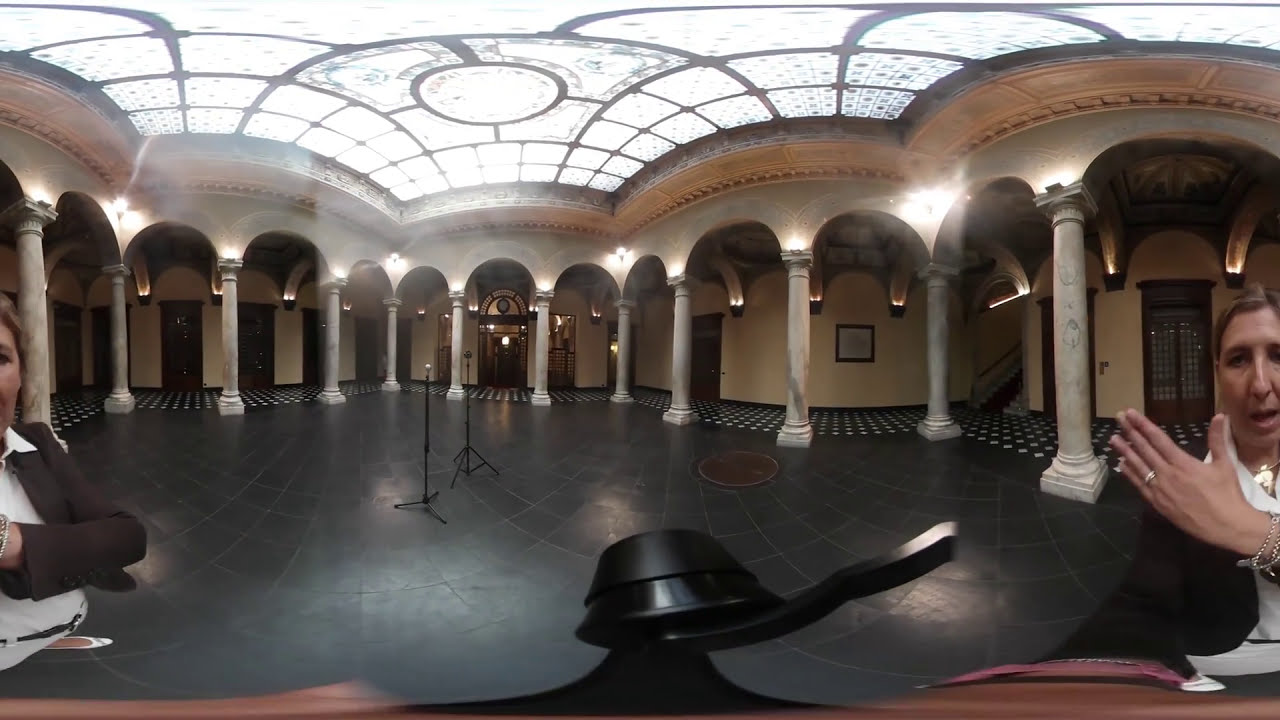The image depicts the interior of a sophisticated building, possibly a museum lobby or a grand hall, characterized by detailed architectural features. The ceiling is adorned with an intricate array of small glass panels, converging into a prominent circular glass panel at its center, permitting light to flood the space. The floor is a polished dark gray tile, seamlessly transitioning to black and white checkered tiles around the perimeter. Surrounding the room, elegant gray pillars stand tall, connected by arches that contribute to the room's grandeur. The far walls are painted a light tan, punctuated by dark brown wooden doors with small glass panels. Notably, two identical women, each wearing a dark brown coat and white collared button-up shirt, are positioned on the left and right, creating a mirroring effect. An upside-down black object resembling a frying pan, and microphone stands are situated in the middle, adding to the room's intriguing layout.